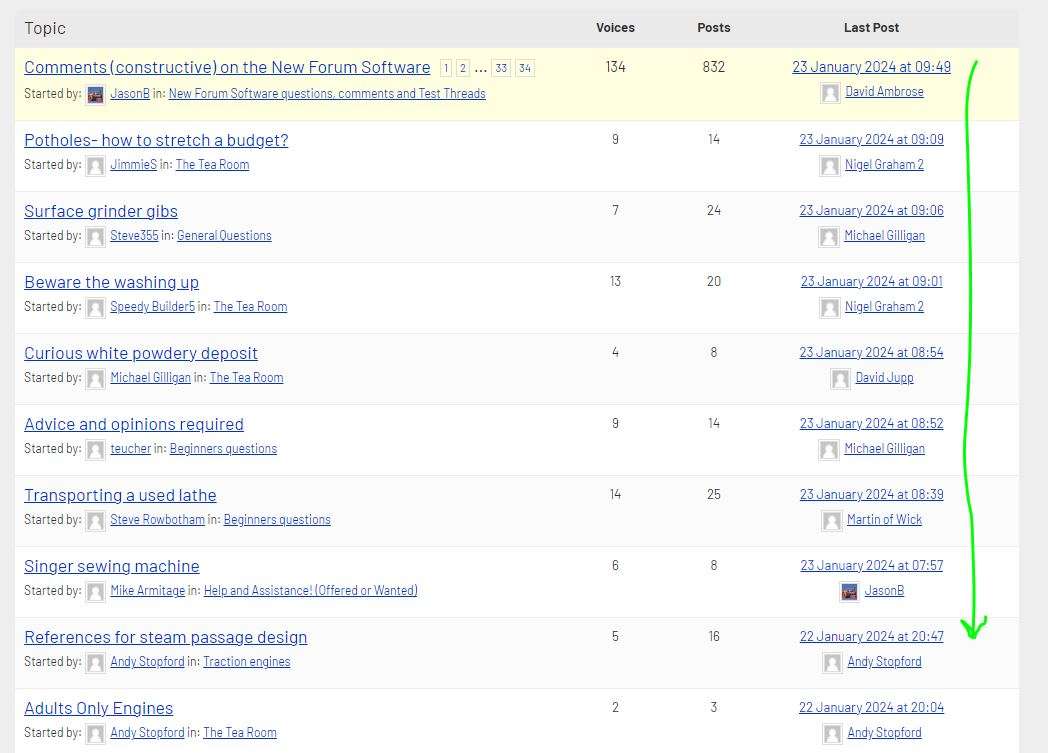This screen capture showcases a structured discussion forum interface, with a gray trim framing both the top and bottom. The top portion features a darker gray strip that houses navigation titles such as "Topic," "Voices," "Post," and "Last Post." Each of these columns appears within the gray interface.

On the leftmost side under "Topics," highlighted in yellow for emphasis, is the top discussion titled "Comments on the New Forum Software," initiated by Jason B. This topic has garnered significant participation with 134 voices and 832 total posts. The latest contribution to this thread was made by David Ambrose on 23 January 2024 at 09:49, using the European date format.

Below this prominent topic are additional discussions including:
- "Potholes"
- "How to Stretch a Budget"
- "Surface Grinder Gibs"
- "Beware the Washing Up"
- "Curious White Powdery Deposit"
- "Advice and Opinions Required"
- "Transporting a Used Lathe"
- "Machine or Sewing Machine"
- "References for Steam Passage Design"
- "Adults Only Engines"

Each of these topics has corresponding last post details, including the date, time, and username of the poster. Adding to the visual details, a green marker arrow is drawn along the right side of the screen, highlighting the column of timestamps for the last posts.

This detailed view provides a comprehensive glance at the forum activity and organization, with clear indication of popular discussions and recent contributions.